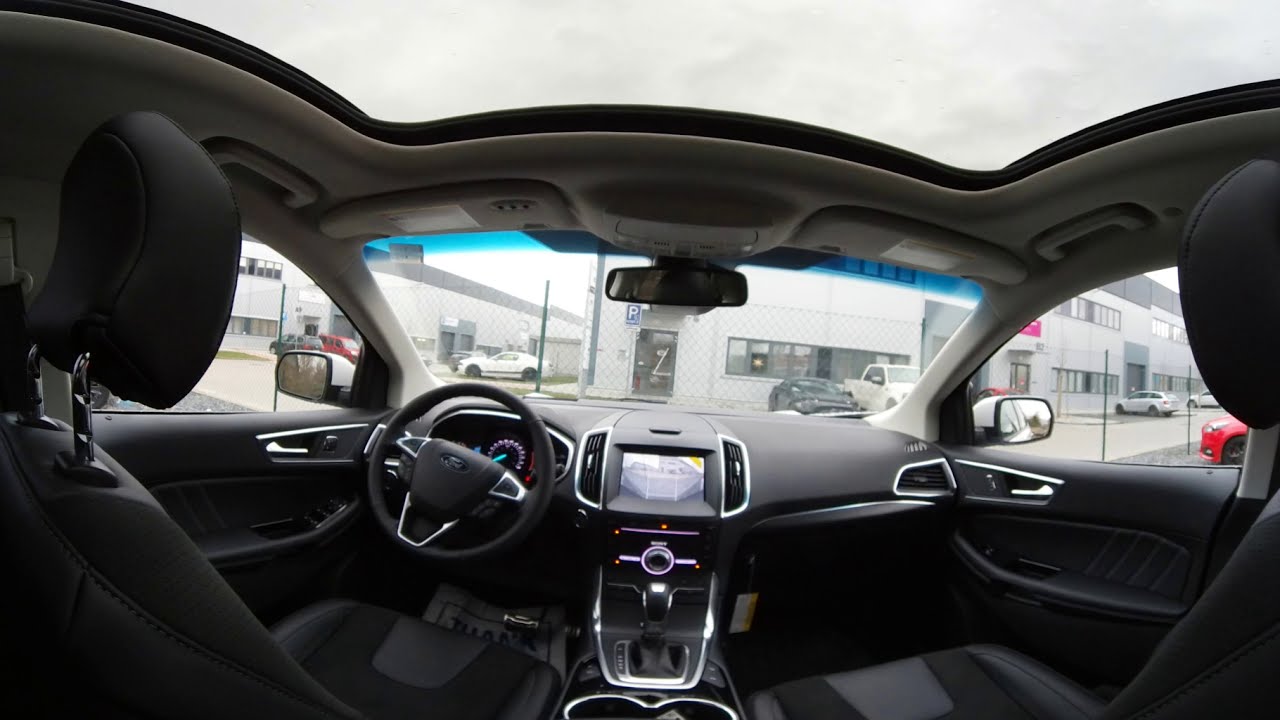From the perspective of sitting in the back middle seat of a newer car with black leather seats, the image captures both the car’s interior and the view outside. The interior features include a TV screen on the dashboard, a clear sunroof revealing a gray sky, and seats upholstered in a combination of deep gray and lighter gray. The dashboard is illuminated with blue, lavender, turquoise, and red lights, and contains a GPS screen among other controls. The steering wheel is on the left-hand side. Through the windows, you can see a white building directly ahead with a 'Z' painted near its door, surrounded by a parking area with a black car and a white truck to the right of the building. Additional buildings flank the main one on the left and right, with several other parked vehicles in front. There is also a parking sign visible among the outdoor scene.